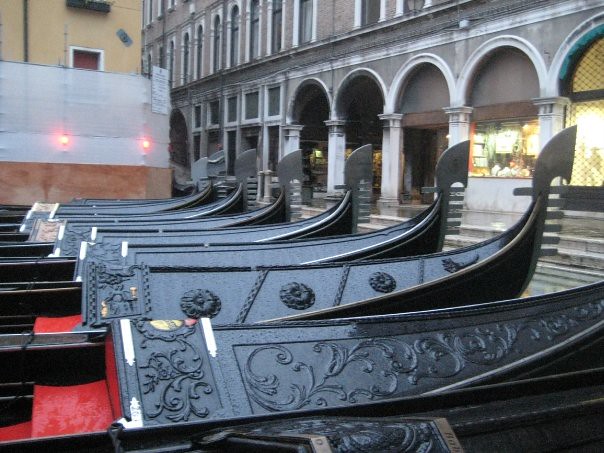The image is set outdoors and showcases a striking scene of sleek, black canoes lined up in the foreground. Each boat is meticulously crafted with red seating areas inside and distinctive decorative designs on the exterior, including swirls, leaves, and floral patterns, some with ornate engravings of round shapes and vines. The boats are made of a black material, possibly metal, and have a unique shape with curled tips and flat fins reminiscent of whale tails. Positioned against the backdrop of an old, tan-colored building, the setting also includes a more prominent, gray structure to the right. This larger building features various rows of windows at the top and a series of arches supported by columns below. The arches form doorways and frame the image's striking foreground elements, combining historical architecture with the elegant artistry of the canoes.